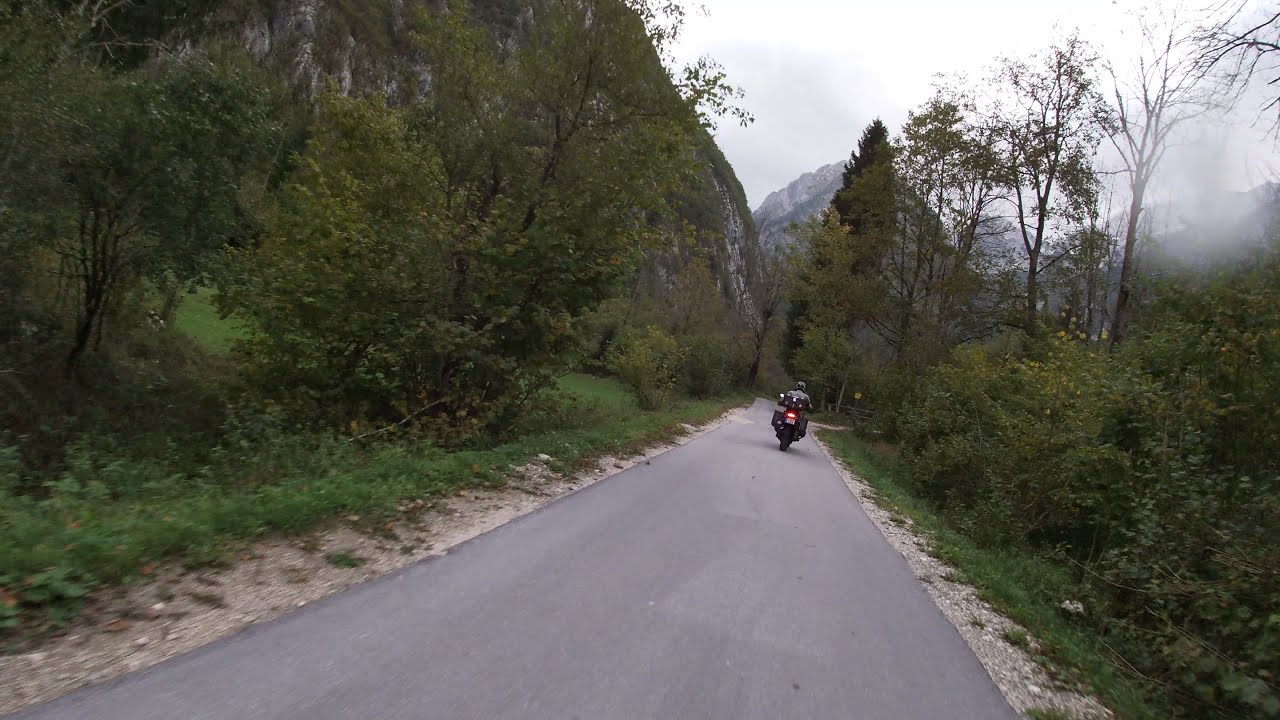The image is a color photograph in landscape orientation, capturing a GoPro video freeze-frame with a point-of-view perspective of a rider on a paved road. The road begins in the lower left corner of the image and shifts slightly towards the center as it extends into the distance. There's no apparent painted lines on the smooth pavement, which appears desolate and infrequently traveled. A motorcycle is visible ahead, roughly 40 yards away, with its brake light illuminated. The rider on this motorcycle is wearing a helmet and the bike is equipped with saddle-like containers. 

The narrow road has a small gravel boundary to the side, which transitions into grass, bushes, and dense trees. These woods flank both sides of the road, with fog predominantly settling in the trees to the right. This scene is set in a mountainous area, suggested by the gray mountain and large cypress tree discernible in the distance. A shroud of mist and fog envelopes the area, partially obscuring the surrounding vegetation and enhancing the sense of high altitude and isolation.